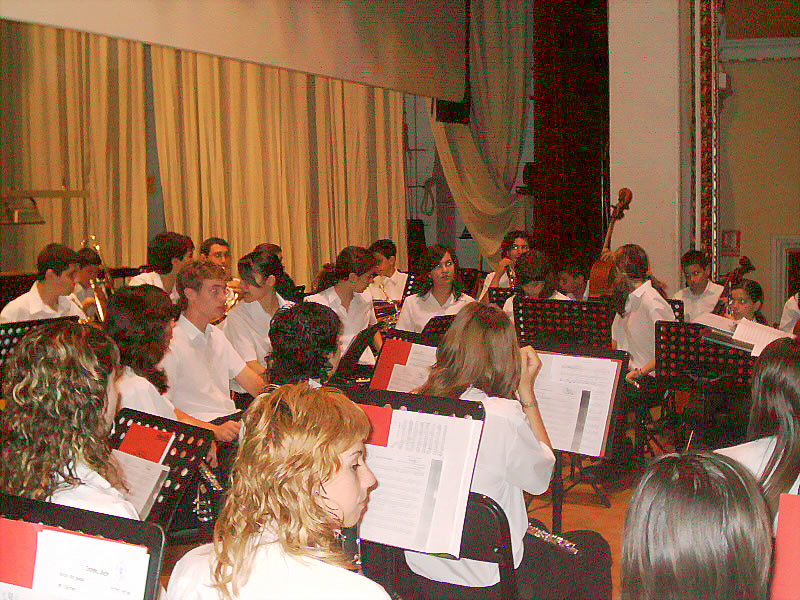This grainy, somewhat pixelated photograph, possibly scanned from an old hard copy, captures a focused group of young musicians who appear to be high school or college age, all of whom are Caucasian. They are arranged in a semicircle formation, seated in dark-colored chairs with black, steel music stands displaying sheets in front of them. Dressed formally, the males in white dress shirts and black pants, and the females in black dresses or white shirts with long skirts, they seem to be engrossed in their music. The ensemble consists of various instruments including flutes, trombones, saxophones, a cello, and a standup bass, indicative of a full-scale orchestra or symphony. They appear to be performing on a stage, as evidenced by the large tan-colored curtain in the background, suggesting a setting within a theater. The central figure, a girl with a flute resting on her lap, adds to the impression of a live music performance.